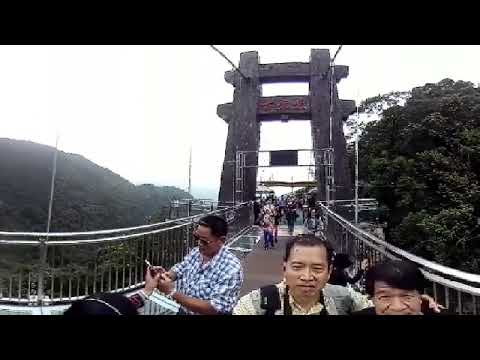The photo depicts a bustling group of tourists on an old bridge, likely set in a mountainous area. The bridge, rectangular and slightly wide, features a distinctive gray metal railing and massive dark brown concrete columns that rise vertically and are connected by two horizontal beams at the top. Cables extending from these beams hint at their structural support role. The background reveals lush green trees on the right and hills on the left, enhancing the scenic beauty under a partly cloudy, blue and white sky.

Up close, three individuals stand prominently; one man, presumably older, has his arm around another, suggesting a familial bond, possibly father and son. They and other tourists, described as being of Asian descent, are casually dressed and equipped with cameras, capturing their moments on the bridge. Some are seen using selfie sticks and phones, indicating a modern-day vacation snapshot. The area appears to be part of a higher elevation, adding to the breathtaking landscape that these tourists are clearly admiring and documenting.